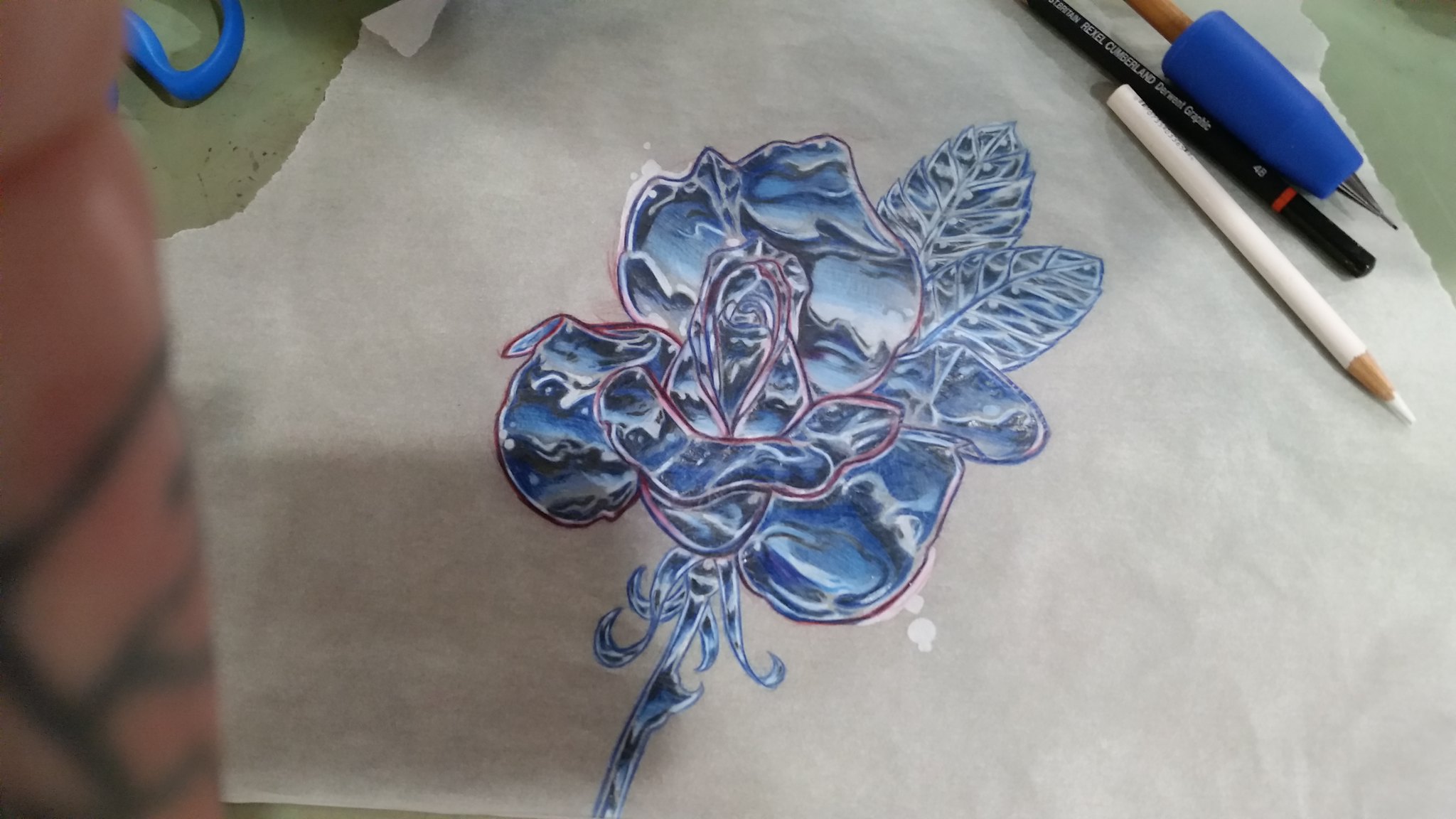In the center of the image, a detailed pre-tattoo flower design is prominently displayed. The flower, resembling a rose, showcases an intricate blend of chrome blues, blacks, and whites, creating a striking metallic effect. The background is speckled with white accents. To the right of the design, a white pencil lies at an angle, suggesting recent use. On the left side, a pair of scissors is positioned next to a hand adorned with tattoos, seemingly belonging to an artist. The hand appears to be involved in the creative process, adding to the authenticity and atmosphere of the scene.